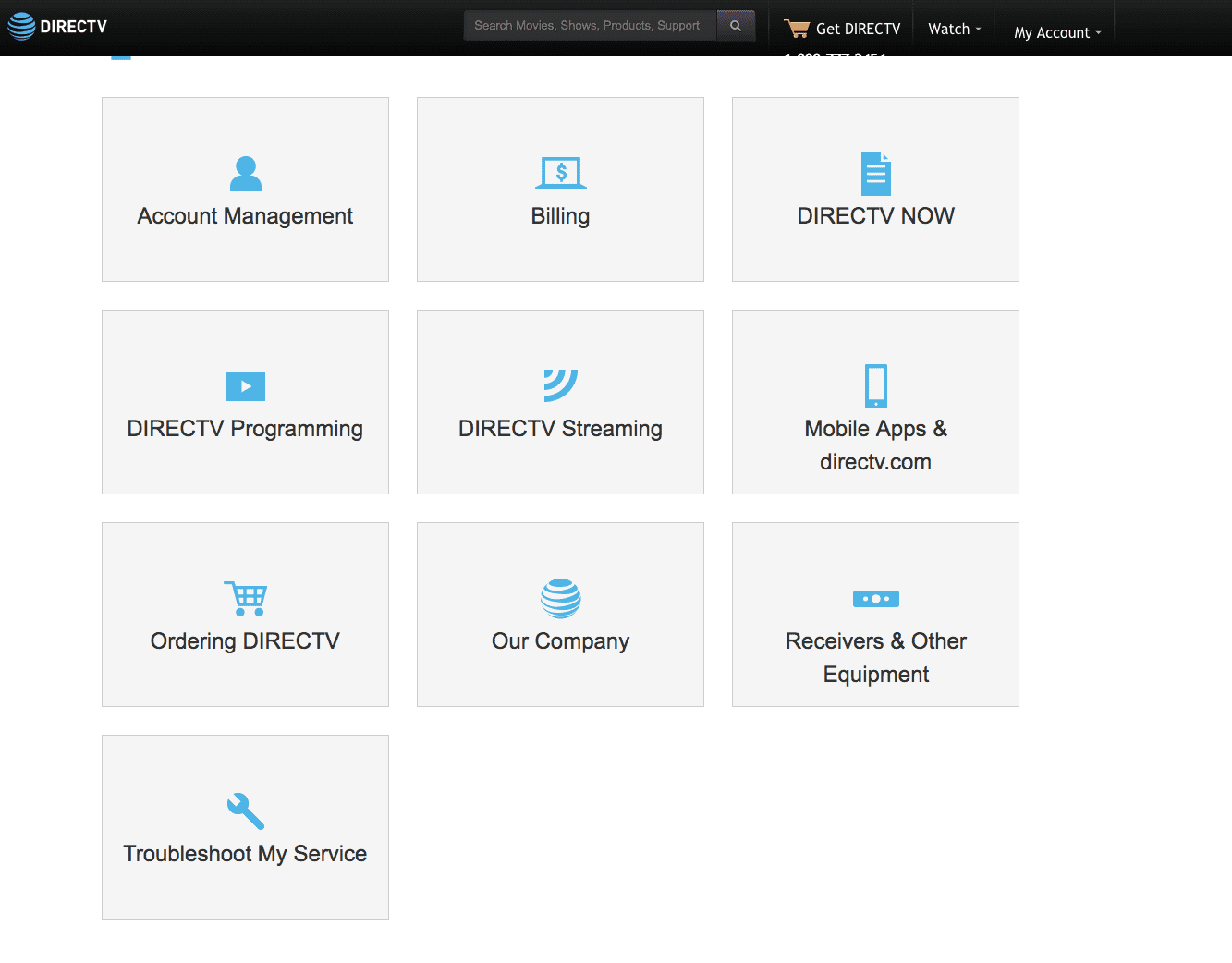Sure, here's a cleaned-up and detailed caption based on the provided description:

---

A screenshot of the DirecTV account management page, featuring elements reminiscent of AT&T's former branding. At the top of the page, a black bar contains a search bar centered within it. Beneath this bar are two pull-down menus labeled "Get to DirecTV - The Yellow Card" and "Watch with," as well as another menu labeled "My Account." The main section of the page has a white background and displays various blue icons within gray boxes, representing different menu options. These options include: Account Management, Billing, DirecTV Now, DirecTV Programming, DirecTV Streaming, Mobile Apps, DirecTV.com, Ordering DirecTV, Our Company, Receipts & Other Equipment, and Troubleshoot My Service. The DirecTV logo, located somewhere on the page, resembles a globe encircled by blue lines akin to the old AT&T logo. The page primarily serves for managing different aspects of a DirecTV account.